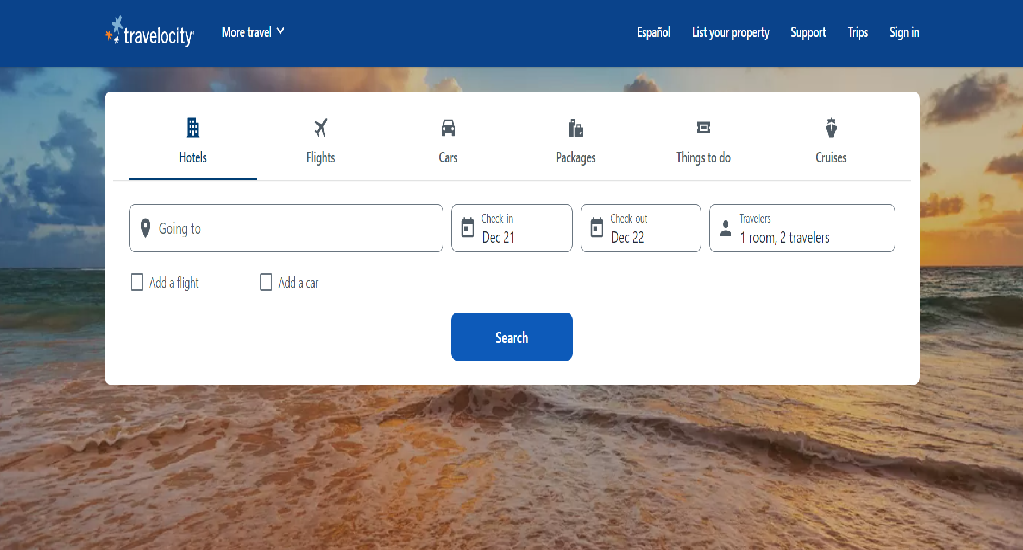The image depicts the Travelocity homepage, designed to facilitate booking travel-related services. The very top of the page features a deep dark blue banner showcasing the Travelocity logo on the far left. To the right of the logo, the words "More travel" are displayed, followed by "Español," "List your property," "Support," "Trips," and "Sign in," all written in white font against the blue banner.

Beneath the banner, the main background image is a stunning ocean view, characterized by deep blue waters and a vibrant sunset, casting orange hues on the water at the bottom. However, much of this scenic picture is obscured by a prominent white search box in the center of the page.

Within this search box are six options, each accompanied by its own icon:
1. **Hotels** - represented by a hotel icon.
2. **Flights** - represented by an airplane icon.
3. **Cars** - represented by a car icon.
4. **Packages** - represented by a package icon.
5. **Things to Do** - the icon for this option is unclear.
6. **Cruises** - represented by a ship icon.

Below these options, the search box is divided into four fields:
1. A large field labeled "Going to."
2. Two smaller fields indicating "Check-in" and "Check-out" dates, listed as December 21st and December 22nd, respectively.
3. A medium-sized field labeled "Travelers," currently set to "One room, two travelers."

Further down, users are presented with two optional check boxes to add a flight and add a car to their booking. At the bottom of the search box, a striking blue button, labeled "Search" in white text, invites users to begin their travel planning.